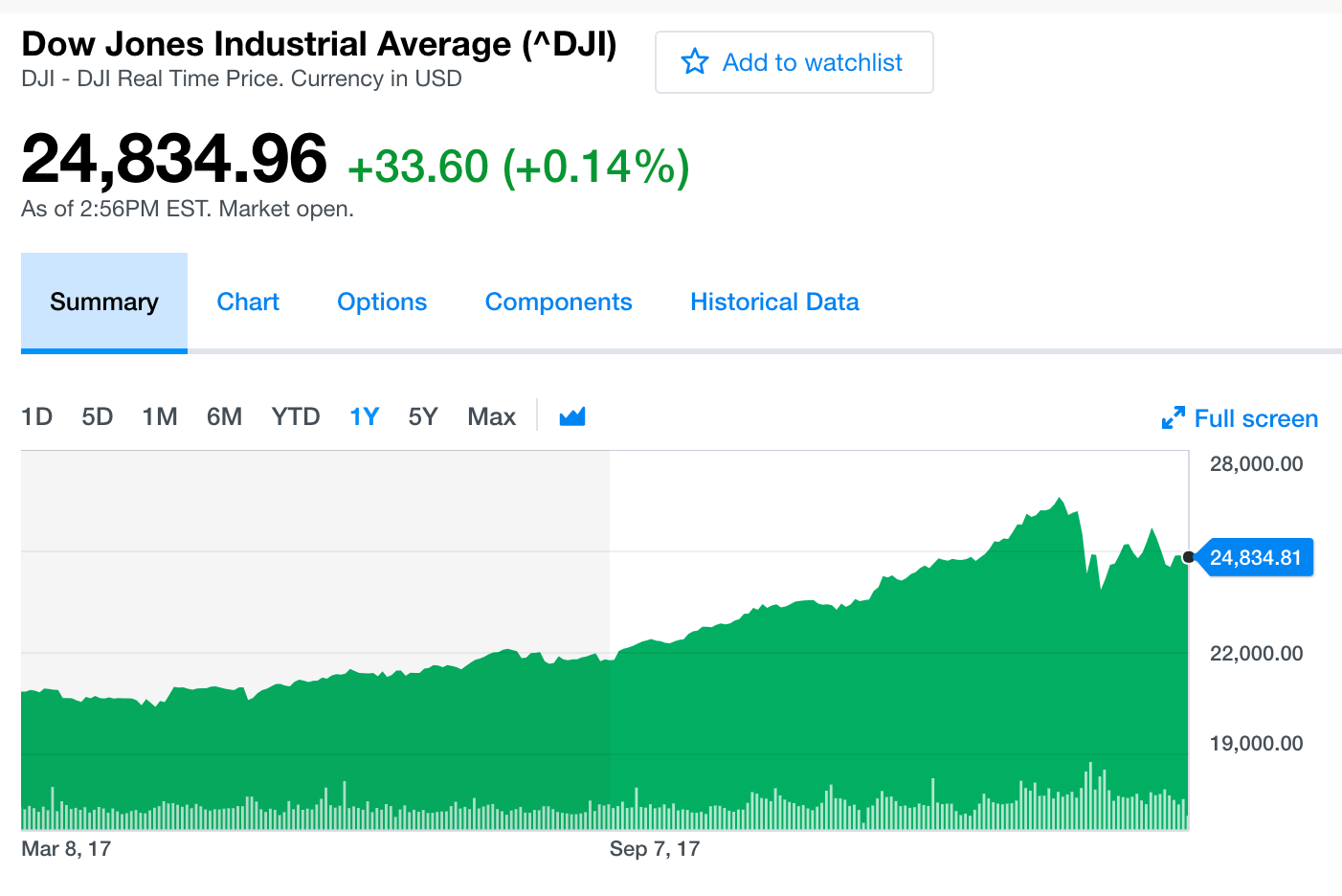The image displays a real-time update of the Dow Jones Industrial Average (DJIA) on a financial website. The index is shown in US dollars, with the current value at $24,834.96 as of 2:56 PM EST. The market is still open, so this value is subject to change. The index has gained 33.60 points, marking a 0.14% increase.

The chart presented is a summary chart, depicting the performance of the DJIA from March 8, 2017, to September 7, 2017. Although the specific data beyond September 7, 2017, is not displayed, the chart provides a clear overview of the highs and lows within the period. The index is performing well, though it's not at its peak.

Additional chart options are available for more detailed analysis, including 'Chart,' 'Options,' 'Components,' and 'Historical Data.' These options offer various timeframes for viewing the DJIA performance: one day, five days, one month, six months, year-to-date, one year, five years, and max duration. The interface also supports a full-screen mode for an enhanced viewing experience.